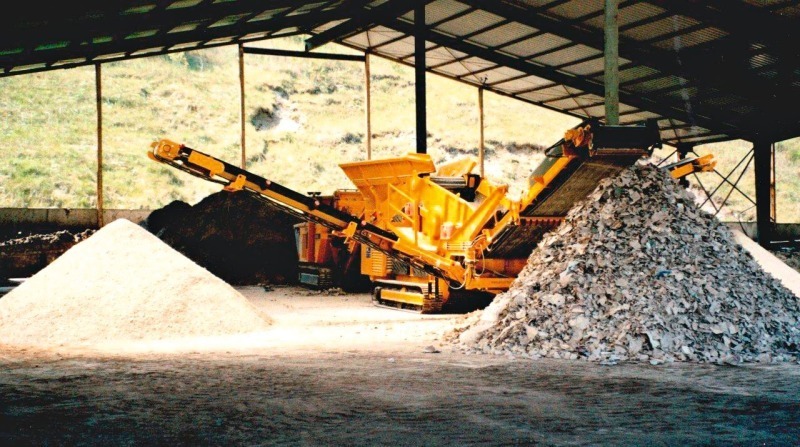In this photograph taken in an open shed area, a large yellow piece of machinery, likely a crusher or recycler, dominates the scene. This machine, equipped with a bay conveyor and two long side arms, is centrally located amid several piles of materials. On the right side and directly behind the machinery is a substantial pile of debris, likely the output from the machine. To the left, there is a smaller pile of fine white powder, possibly crushed sand or rocks, and another darker brown pile closer to the machine. Green supports uphold the shed's roof, which features black girders with white panels in between. The background reveals a hillside covered in green vegetation, visible through the open sides of the shed.